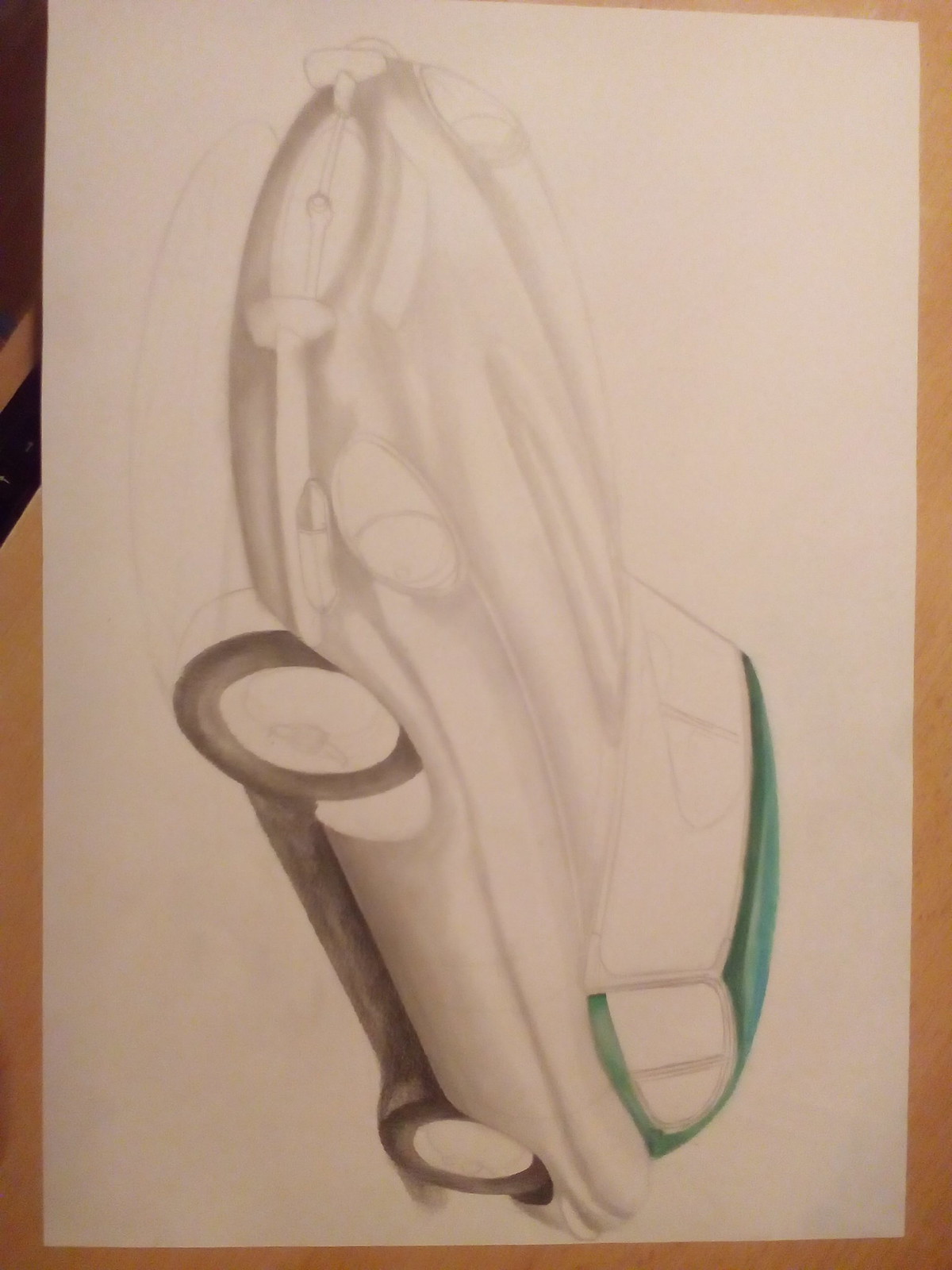This image features a detailed pencil sketch of a vintage sports car, likely from the 1970s, drawn on a basic white piece of paper. The sketch showcases the car from a side view and includes heavy use of shadows to suggest depth, particularly beneath the car, enhancing its three-dimensional appearance. The tires are distinctly shaded in black. The car’s hood stands out with its gradient of green hues, transitioning from a blue-green to a light green and then to a darker green, while the rest of the car maintains a soft, gray pencil tone. The background depicts a light honey brown wood table, adding a subtle contrast to the gray and green of the sketch.